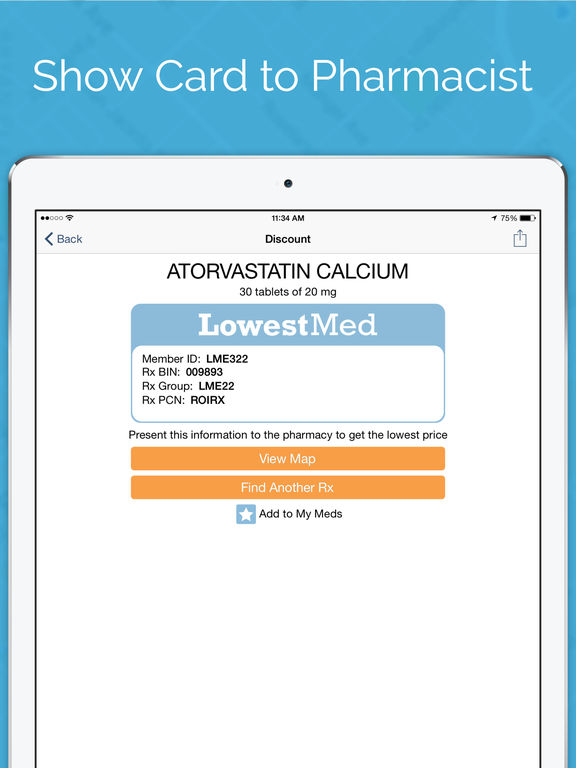A large blue poster prominently displays the message "Show card to pharmacist." The poster features the image of a white Apple iPhone with a timestamp of 11:34 AM, a battery level at 75%, and an open app showing a discount offer. Users have the option to either go back or download the discount. Below the phone image, there's information about Atorvastatin Calcium, a medication available in 30 tablets of 20 milligrams each. Key details such as the member ID number, prescription BIN number, prescription group number, and prescription preferred network are displayed within a boxed area. An instruction reads, "Present this image with this information to the pharmacy to get the lowest price." The poster also includes an orange bar labeled "View map," which users can click on, and another orange bar labeled "Find another prescription." At the bottom, there is a starred button titled "Add to my meds." The overall message suggests that the app helps users get the lowest possible price for their prescriptions, specifically for Atorvastatin Calcium in this case.